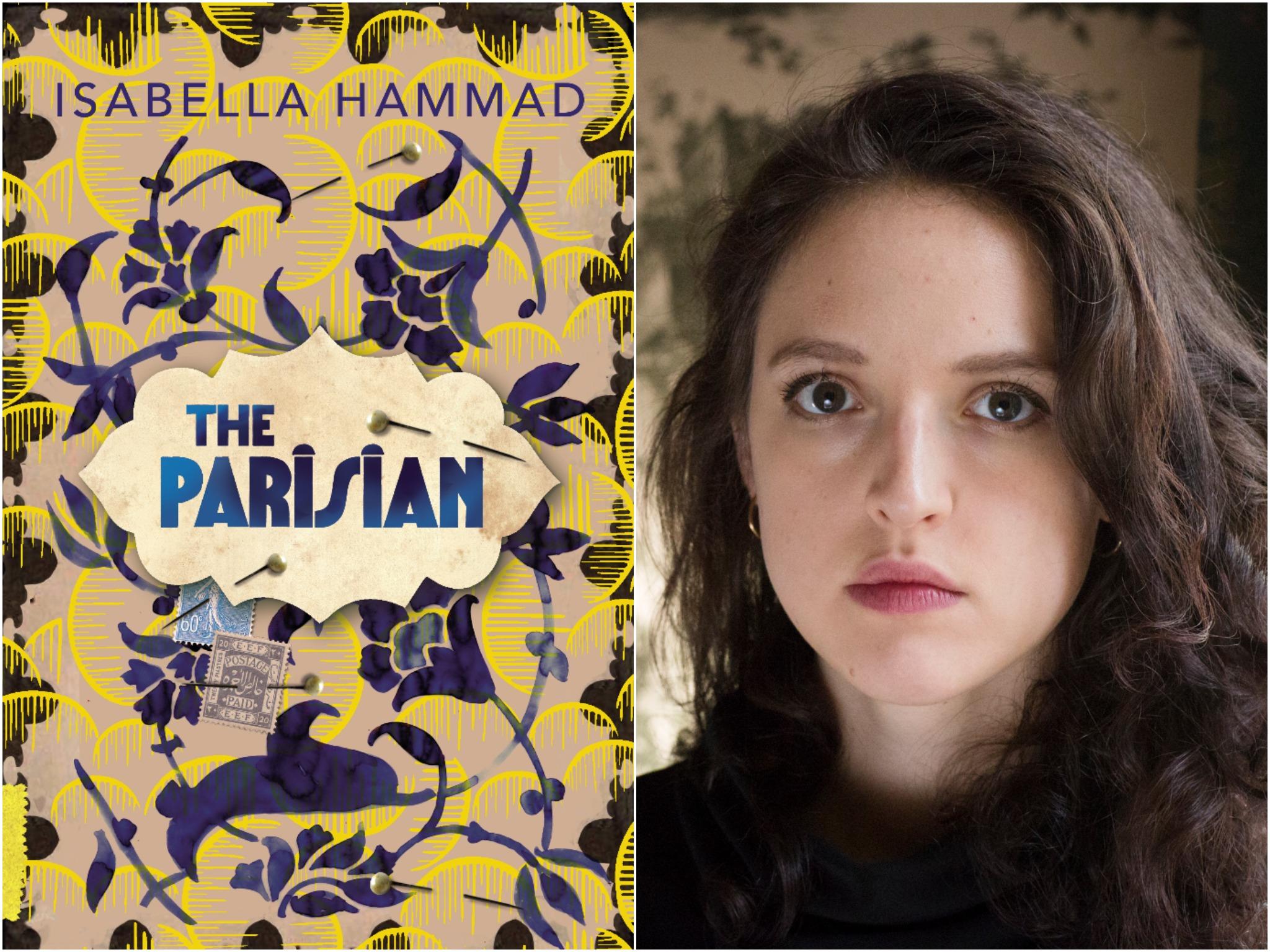This image features a side-by-side collage comprising a book cover and a portrait, likely of the author. The left side displays the cover art for "The Parisian" by Isabella Hamad, with her name gracing the top. The intricate design of the cover is dominated by a vivid palette of blue and yellow. The background contains abstract patterns of blue flowers and yellow crescent shapes, some adorably textured with vertical lines. The book title is set in blue text within a decorative, cloud-like plaque, secured with two pins and accompanied by stamp-like illustrations marked "Postage Paid." The right side presents a serious-looking young woman, presumably Isabella Hamad, with long, wavy dark brown hair and dark eyes. She wears pink lipstick and gazes directly at the camera. The backdrop behind her is light tan or off-white wallpaper adorned with green plant motifs.